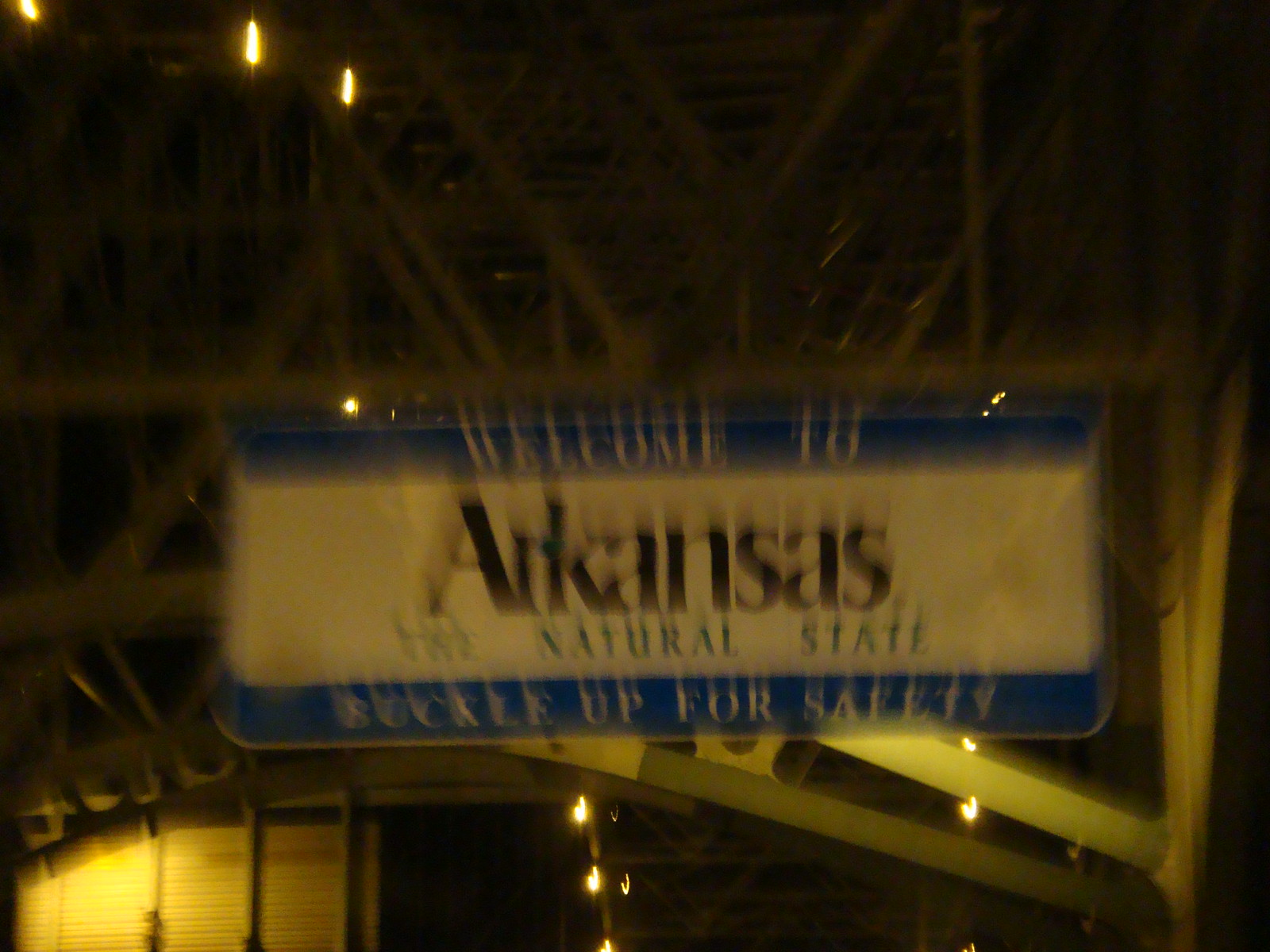This photograph appears to be taken at night from a moving vehicle crossing a bridge. The bridge features distinct white elements and diverse architectural designs, illuminated by lights. A prominent, albeit blurry, blue and white sign reads, "Welcome to Arkansas, the natural state, buckle up for safety," with "Arkansas" highlighted in black. The motion blur suggests the vehicle was in transit when the image was captured, adding a dynamic sense of movement to the scene.